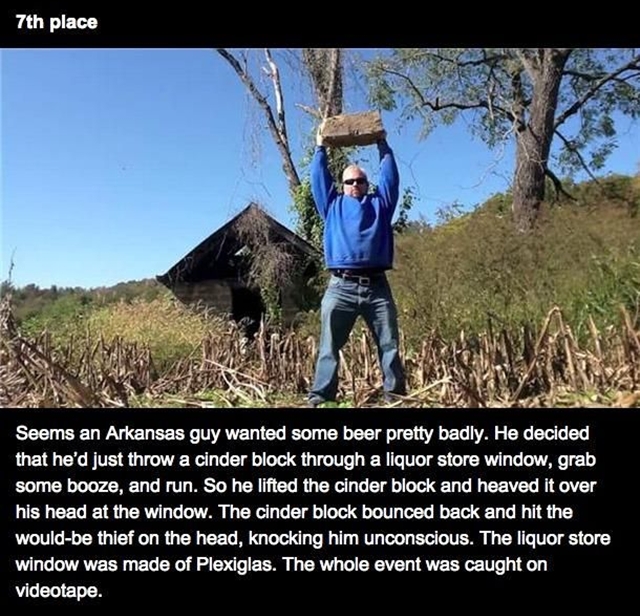The image depicts a man standing in a field of dried grass, holding a cinder block above his head with both hands. He is wearing a blue sweatshirt, blue jeans, and sunglasses, and has blonde hair. In the background, there is a wooden house and some trees. The setting suggests an outdoor area with evidence of deforested land, as tree stumps and sticks are visible. The top left corner of the image displays the text "7th place" in white letters on a black background. At the bottom, white text against a black background reads: "Seems an Arkansas guy wanted some beer pretty badly. He decided that he'd just throw a cinder block through a liquor store window, grab some booze, and run. So he lifted the cinder block and heaved it over his head at the window. The cinder block bounced back and hit the would-be thief on the head, knocking him unconscious. The liquor store window was made of plexiglass. The whole event was caught on videotape."